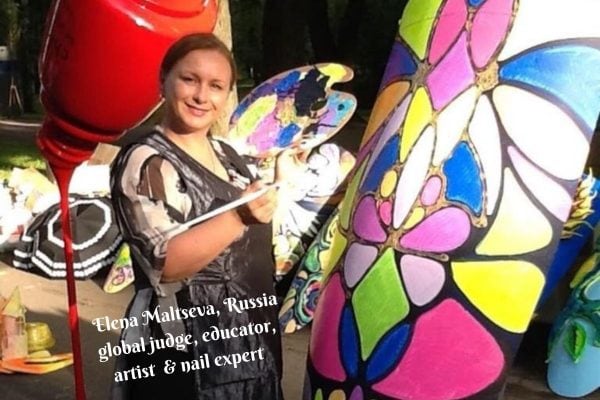In this vibrant and detailed collage-style photograph, we see Elena Maltseva, a distinguished Russian global judge, educator, artist, and nail expert, standing on the left side of the image. Dressed in a black apron over a black and white shirt and black pants, she holds a messy paint palette in her left hand and a paintbrush in her right. Elena is caught in a poised stance, gazing directly at the camera. 

To her right, an enormous, intricately designed pillar rises, adorned with patterns in hues of yellow, pink, blue, white, light purple, and black, resembling flower petals or a butterfly design. Above her, an oversized inverted bottle, likely part of an art exhibit, pretends to pour streams of red paint, adding a whimsical touch to the scene. Accompanying this rich visual display is superimposed text near the bottom left, angled elegantly, that reads: "Elena Maltseva, Russia, global judge, educator, artist, and nail expert." This photograph masterfully blends elements of a live art exhibit with digital graphic design, capturing the creative energy and expertise of Elena Maltseva.